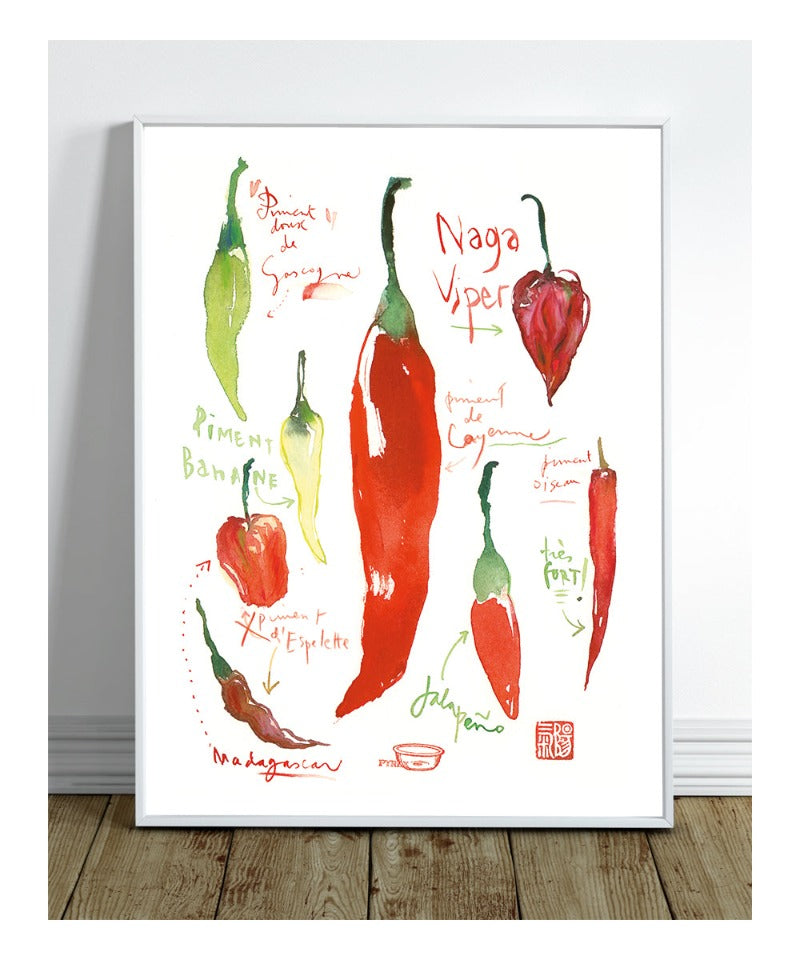This vertically rectangular poster, framed in white, is leaning against a grayish-white wall with a wooden floor beneath it. The poster, set against a white background, features artistic watercolor illustrations of various peppers, each labeled with its name. In the center, prominently displayed, is a red cayenne pepper labeled "Piment de Cayenne." Surrounding it are peppers of different types: to the left, a green pimento; below it, a yellow banana pepper ("Piment Banan"); beneath that, a red pepper labeled "Piment d'Espelette"; to the right, a long, curly red pepper called "Madagascar"; in the top right corner, a red, heart-shaped "Naga Viper"; a long red jalapeño named "Jalapeño"; and a slim red pepper labeled "Piment d'Oiseau," which translates to "bird pepper" and has the note "très fort" ("very strong") beside it. An artist's signature adorns the bottom left of this visually appealing and informative poster.